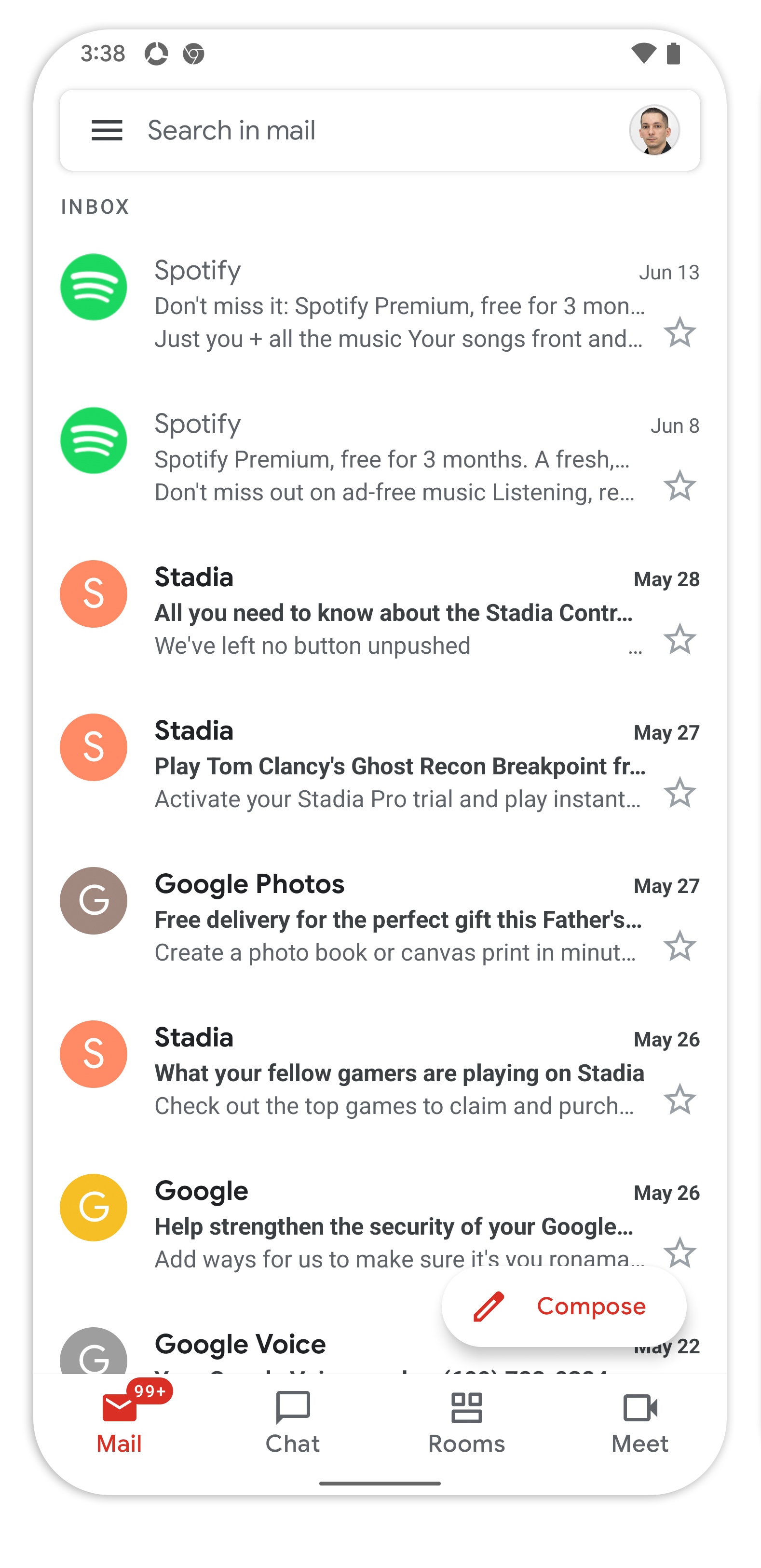**Caption:**

A screenshot captured at 3:38 on a smartphone, displaying the email inbox. The search bar at the top reads "Search in mail." Below the search bar is the inbox, featuring various promotional emails. The first email snippet mentions "Spotify" multiple times, highlighting offers for "Spotify Premium free for three months" with mentions of music and personal songs. Following that, another email from Spotify reiterates the same offer, emphasizing ad-free music listening.

The third email snippet refers to "Stadia," possibly mentioning an informational content about Stadia with "all you need to know about the Stadia..." text, indicating thorough coverage with the phrase "we've left no button unpushed." 

Subsequent emails from Stadia include mentions of "Tom Clancy's Ghost Recon Breakpoint" inviting users to "activate your Stadia Pro trial" for instant play access. Finally, there is an email from Google Photos promoting "free delivery for the perfect gift this Father’s Day," aiming to entice users with timely celebratory options.